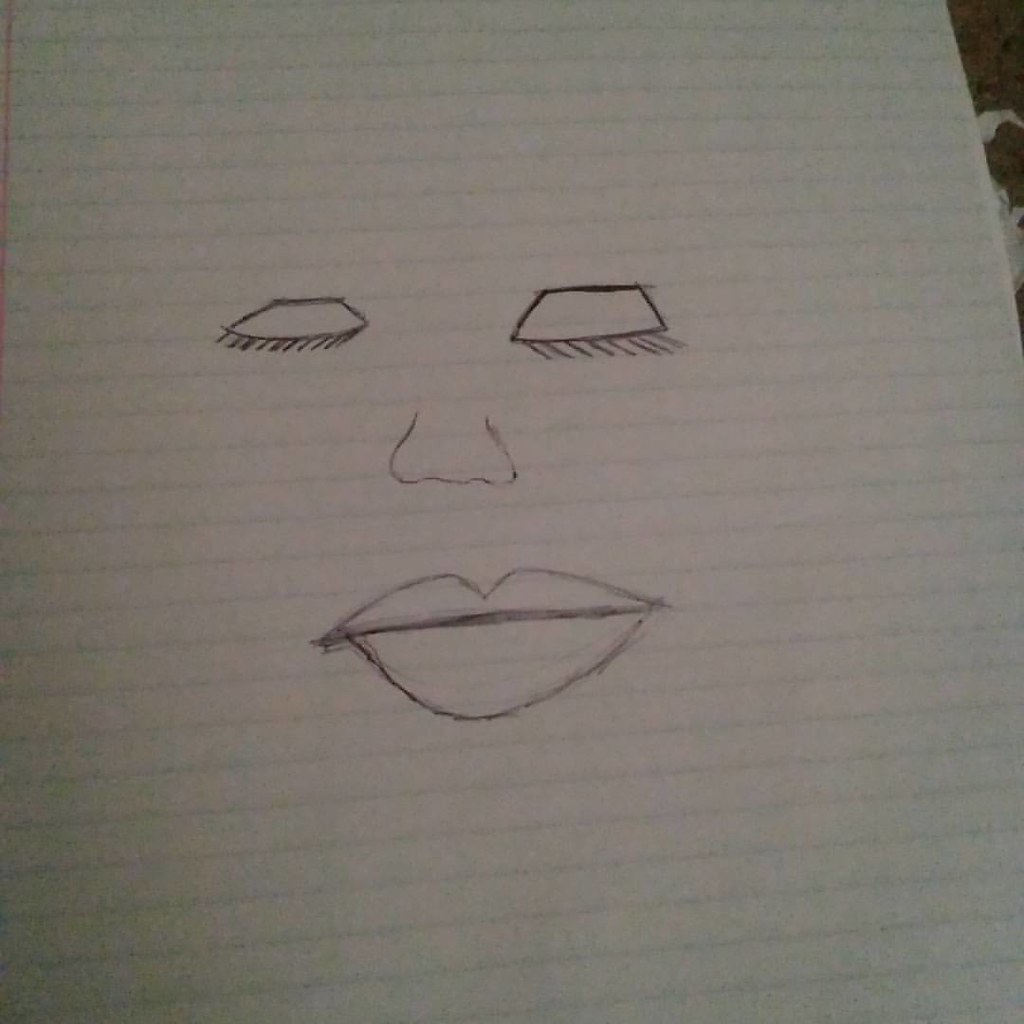This is a simple yet detailed doodle on a piece of lined notebook paper, depicting only facial features. In the center of the page are two closed eyes, each drawn with eyelids shaped like trapezoids. The eyes are adorned with numerous eyelashes; the left eye's lashes extend downwards to the left, while the right eye's lashes extend downwards to the right. Beneath the eyes, there's a wider set nose, resembling the shape of an 'L' followed by an upside-down 'U', another upside-down 'U', and a backward 'L'. The lips are quite full, with the bottom lip noticeably larger. The top lip is drawn with a subtle curve, creating a delicate rosebud shape, and there's a thick line defining the middle of the lips. The drawing lacks a complete head, focusing solely on these facial elements and utilizing the horizontal lines of the paper for alignment and structure.